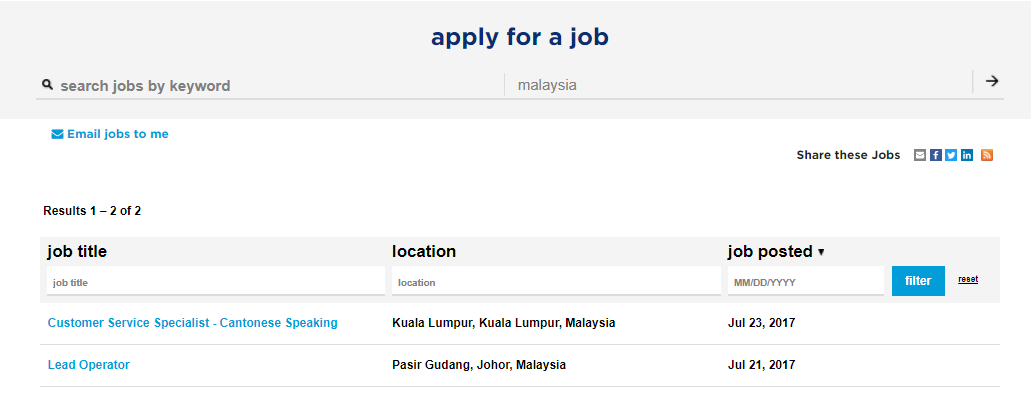The screenshot displays job listings on a website. The interface is more horizontally oriented than vertically. A gray banner at the top prominently features the text "Apply for a job in Blueprint." Directly below the banner is a search bar with a black magnifying glass icon and placeholder text in gray, reading "Search jobs by keyword."

To the right of the search bar, the text "Malaysia" is displayed alongside a black arrow pointing to the right. Below this section, there is an option labeled "Email jobs to me" accented by a blue clickable button. Additionally, options to share job listings through various platforms, including email, Facebook, Twitter, Indeed, and an unidentified orange icon, are available.

The central section of the screenshot indicates that there are "Results 1-2 of 2." This area includes column headers for job title, location, and date posted, each accompanied by drop-down filter menus, a blue "Filter" button, and a "Reset" button for adjustments.

Two job listings are displayed in blue text:

1. **Customer Service Specialist (Cantonese Speaking)**
   - Location: Kuala Lumpur, Kuala Lumpur, Malaysia
   - Date Posted: July 23, 2017

2. **Lead Operator**
   - Location: Pasir Gudang, Johor, Malaysia
   - Date Posted: July 21, 2017